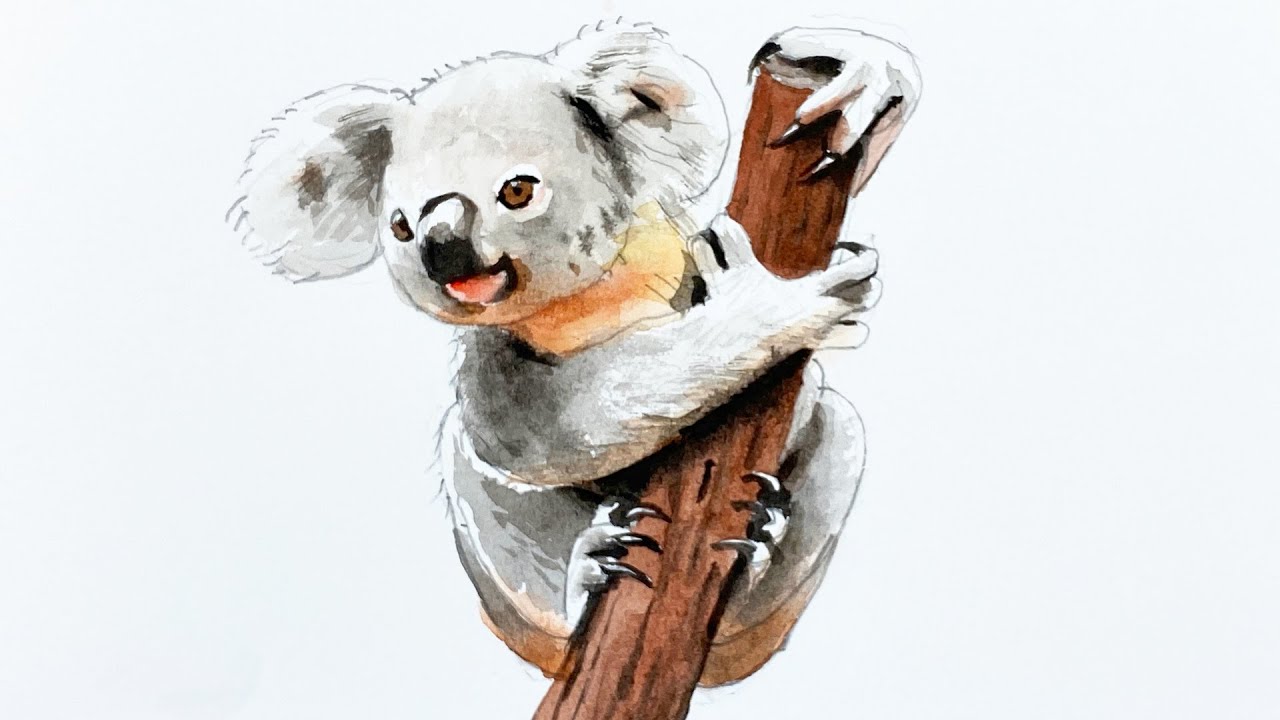This image features a detailed watercolor painting of a baby koala bear clinging to a tree branch. The koala, primarily white with gray patches and tints of tan around its neck and bottom, displays immense detail in its claws and feet, which are grasping onto the brown, leafless branch. One hand is positioned atop the branch while the other curls around it, visible with sharp, long nails. The koala's big brown eyes look contemplative, and its opened mouth reveals a tiny pink tongue, suggesting it is panting. The background is a subtle bluish-gray, adding a serene contrast to the vivid detailing of the bear and branch. This artwork captures the tender and earnest expression of the young koala, highlighted by its large ears and distinct black nose.